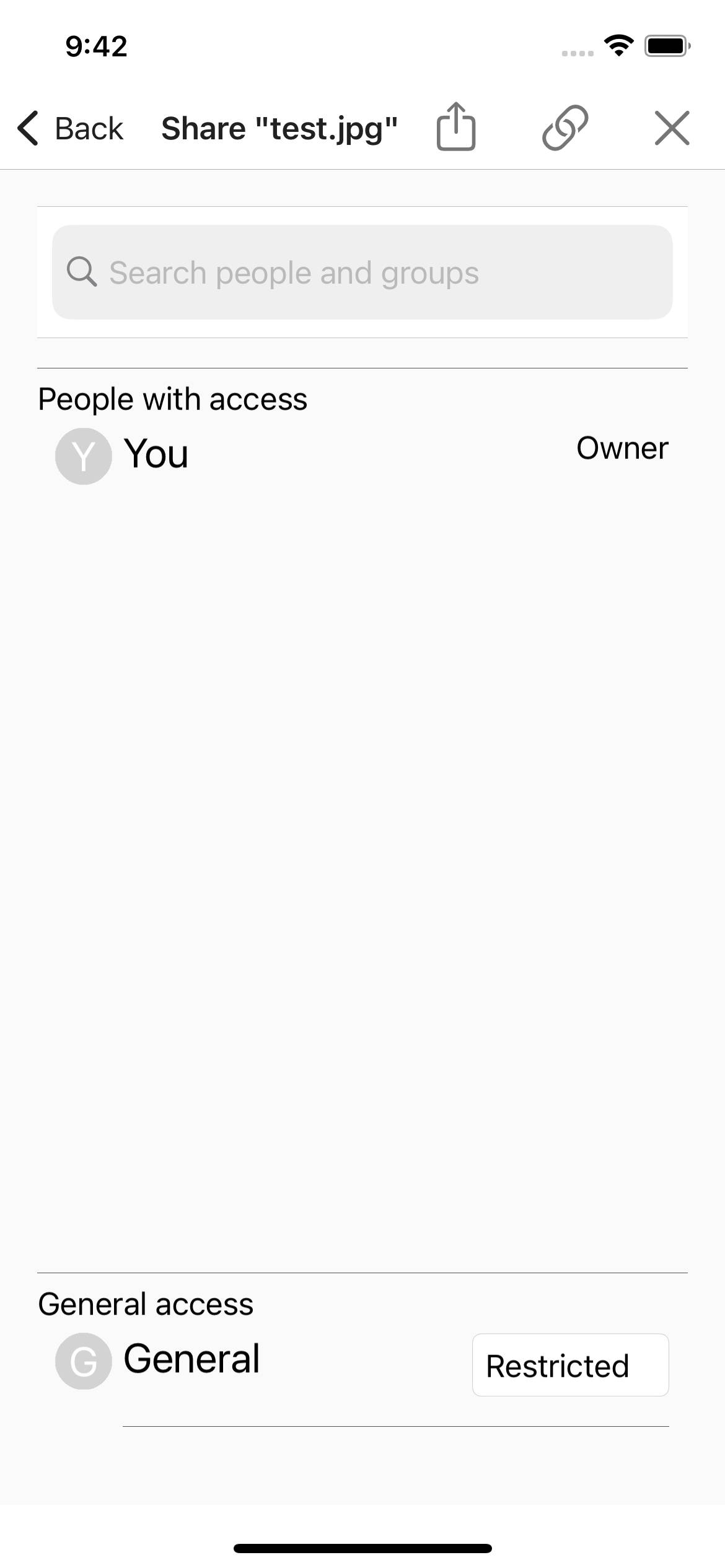Screenshot of a Mobile Phone Interface - Detailed Description

The image depicts a mobile phone interface, specifically a webpage or search result. 

- **Top Status Bar**: 
  - At the upper left, the time displayed is 9:42.
  - On the right, there are multiple icons: 
    - Four horizontal dots
    - Wi-Fi signal icon
    - Battery icon which shows full charge.

- **Navigation Bar**: 
  - Below the status bar, there is a navigation bar with several options:
    - "Back" with a left-pointing arrow
    - "Share" option
    - The text "test.jpg" enclosed in quotes 
    - An icon resembling a file upload icon 
    - An icon resembling a link of a chain 
    - An "X" icon.

- **Search Bar**: 
  - Under the navigation bar, there is a search bar in a grayish-blue rectangle with the prompt "Search people and groups" and a magnifying glass icon.

- **Access Information**: 
  - Below the search bar, the section titled "People with access":
    - The word "You", preceded by a "Y" in a bluish-gray circle
    - To the right of "You," it states "Owner".

- **General Access**: 
  - At the bottom, there is a section titled "General access":
    - The word "General" with a "G" in a grayish-blue circle
    - A rectangle to the right that says "Restricted".
  - The interface concludes with a black horizontal line at the bottom.

This detailed description captures the specifics and layout of the mobile phone interface, providing a clear and structured view of the elements present in the screenshot.